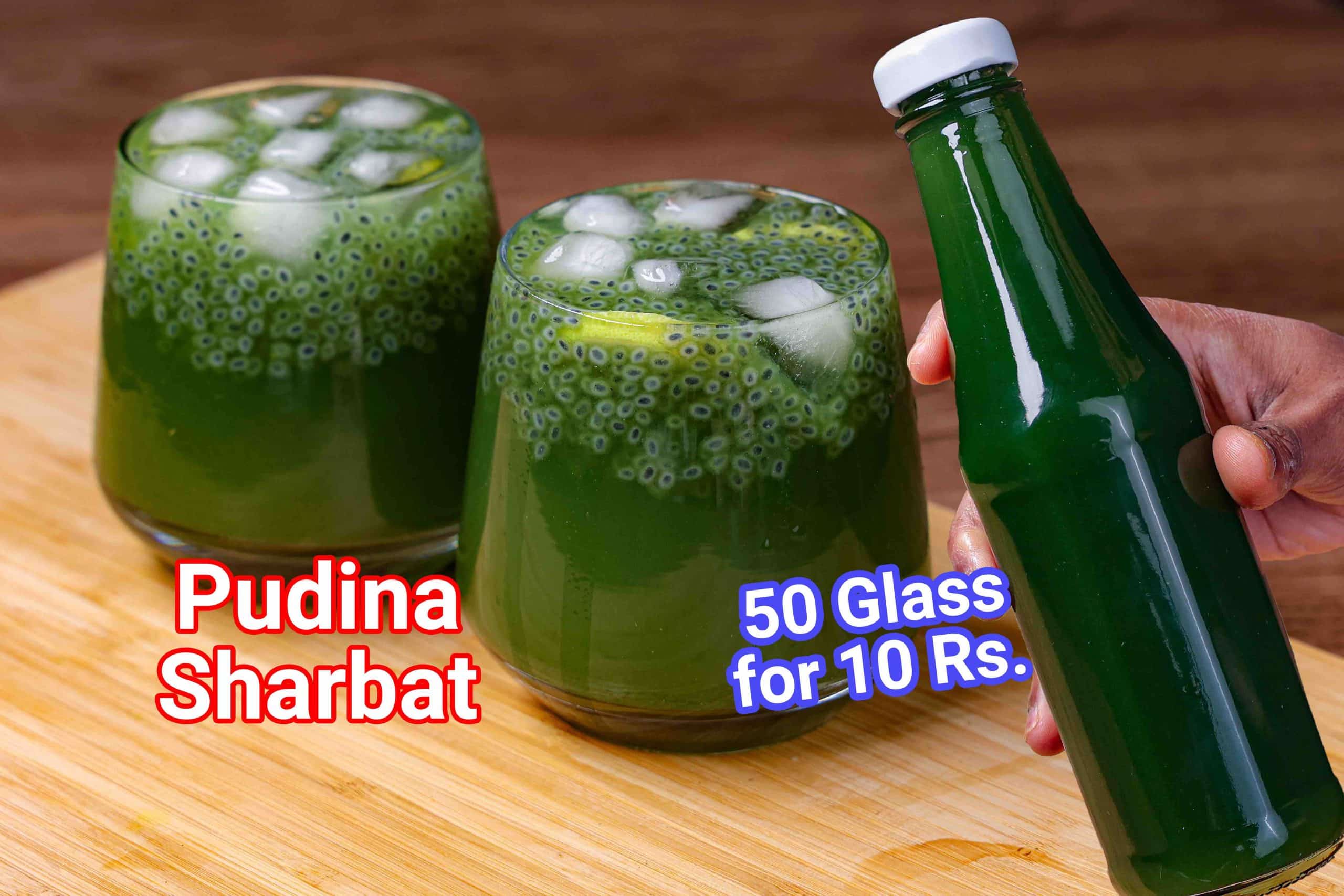The image depicts a vibrant scene featuring two short glasses filled to the rim with a green liquid, likely Pudina Sharbat. The drinks contain ice cubes and possibly slices of lemon or lime. Suspended within the liquid are tiny white, circular seeds, which may be chia seeds. A brown-skinned hand is holding a glass bottle with a white cap, containing the same green concoction without the ice. The setting is atop a light brown cutting board, and the background appears to be a brown, wooden surface. Text in the image indicates that the drink is Pudina Sharbat, with a promotion offering '50 glasses for 10 RS' in white font outlined in red and purple. The overall scene appears to be an advertisement for this refreshing beverage.